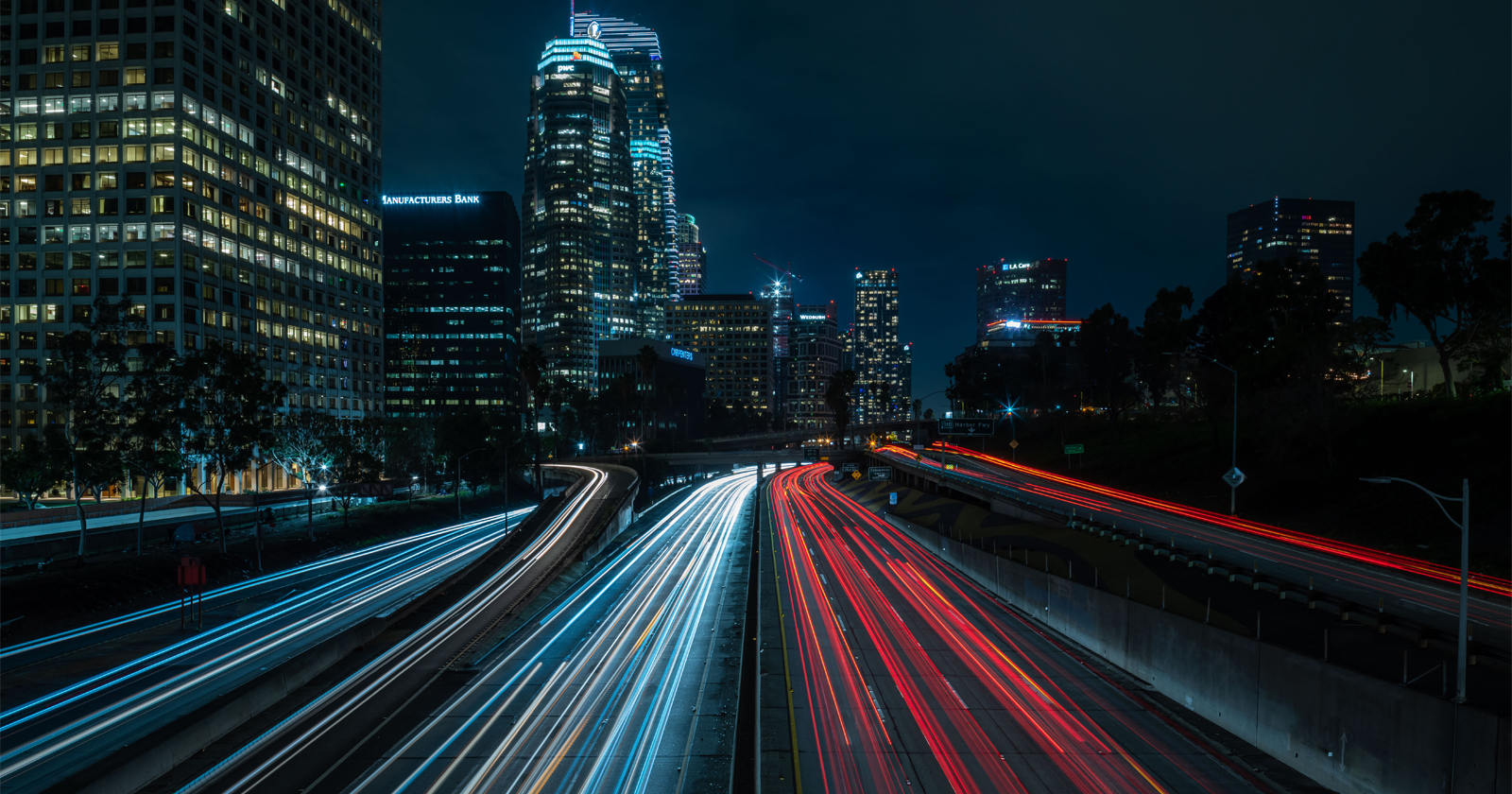This photograph captures a bustling cityscape at night, with a dark sky painted in shades of blue and black. Towering skyscrapers and apartment complexes dominate the background, their numerous windows sporadically illuminated. One prominent building proudly displays "Manufacturers Bank" in glowing blue and white letters. The image artfully showcases the hurried pace of city life, with a highway or bridge running through the center. The road is animated with streaks of white and red lights left by moving vehicles, creating a dynamic and almost painterly effect. In the foreground on the left, there's a row of trees silhouetted against the backdrop, while to the right, a body of water subtly reflects the ambient lights. Despite the absence of active streetlights, the scene is vibrant with the shimmering lights from the buildings and the flowing, streaky car lights that create an enchanting, almost surreal atmosphere.